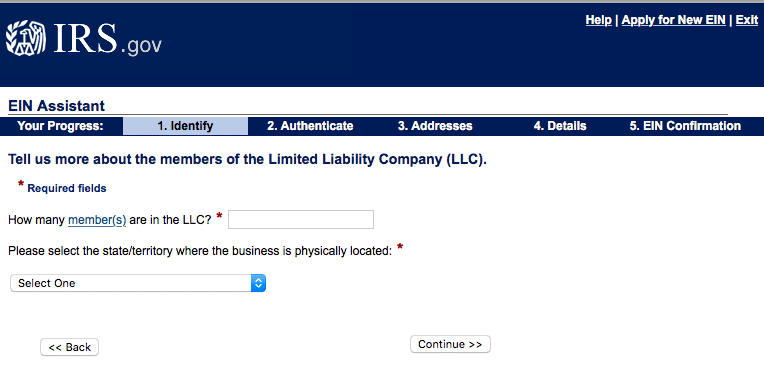The image depicts a webpage from the IRS website, specifically a section for applying for a new Employer Identification Number (EIN). The browser tab reads "Help Apply for New EIN – Exit," indicating this is part of a step-by-step application process. The process includes five steps: Identify, Authenticate, Addresses, Details, and EIN Confirmation.

The user is currently on the first step, "Identify," which involves providing details about the members of a Limited Liability Company (LLC). The step is clearly labeled with instructions to "Tell us more about the members of the Limited Liability Company (LLC)" and includes a red asterisk to denote required information. The two main questions on this page are: "How many members are in the LLC?"—with "members" being an underlined, clickable term—and "Please state the state/territory where the business is physically located."

Navigation buttons labeled "Back" and "Continue" are situated at the bottom of the page. The webpage design prominently features a very dark, almost midnight blue color, with text frequently contrasting in white for better readability. The current step, "Identify," displays its text in black, whereas the titles for the other steps are presented on a dark blue background with white text.